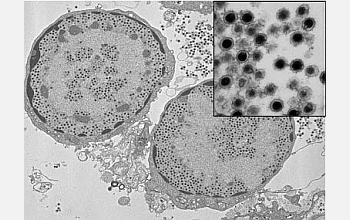The image depicts a scientific scene resembling what one might observe under a microscope, rendered in black and white. It appears to be meticulously hand-drawn, possibly with pencil. The image is rectangular with off-white or light gray borders and a gray background. The central part of the composition features two large, round cell-like structures surrounded by numerous small dots along their perimeters. These dots give texture and detail to the cells. In the upper right corner, there's a picture-in-picture element—a square with a black border containing a dense cluster of small black and gray spots, suggesting a zoomed-in view of one of the cells. The detailed and textured depiction evokes a microscopic slide one might study in a laboratory or science class, hinting at the exploration of bacteria or similar microorganisms.